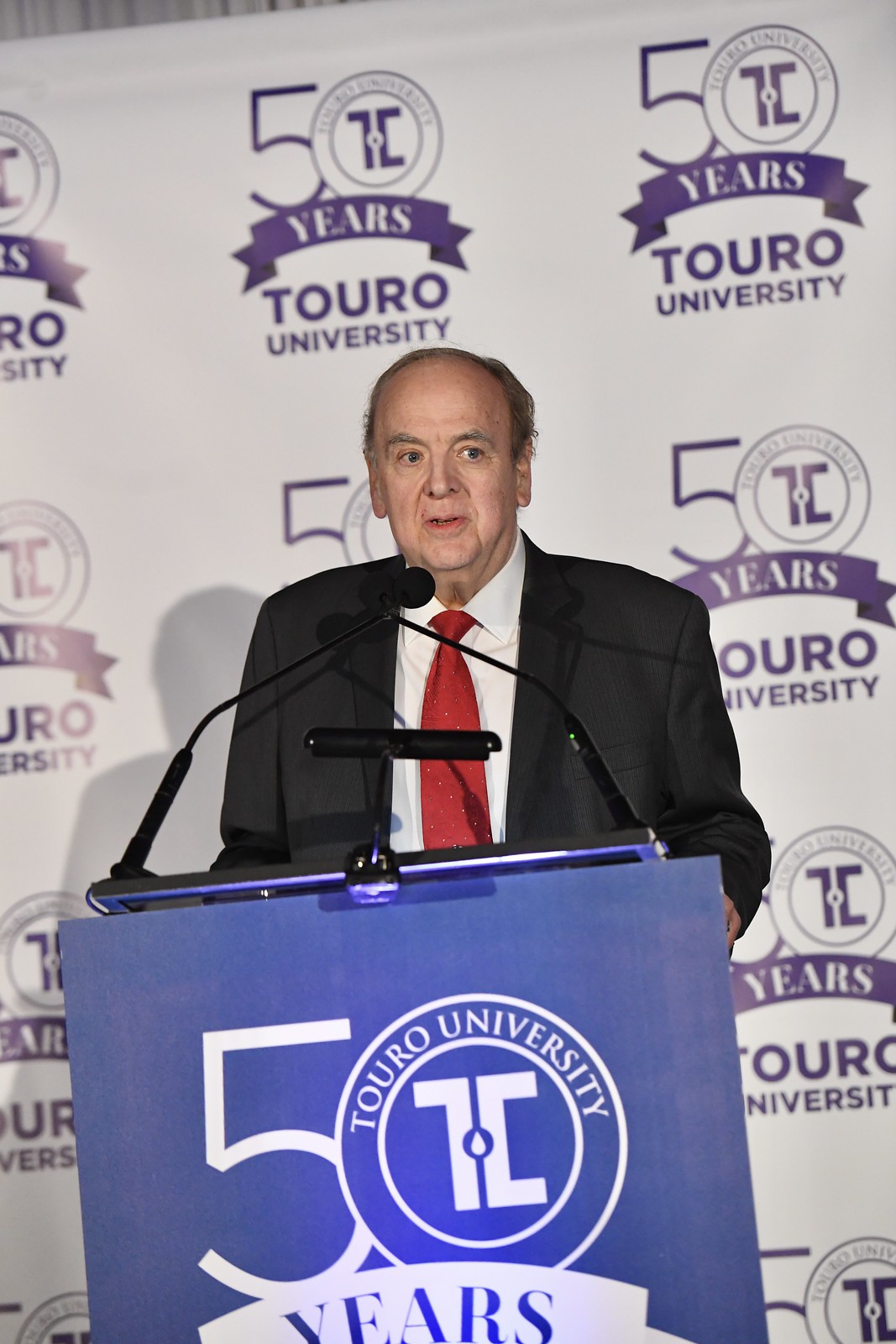In the image, an elderly man stands at a blue podium adorned with multiple microphones, delivering a speech at a notable event celebrating 50 years of Touro University. He is dressed in a typical black suit, complemented by a white shirt and a red tie. The podium prominently features the Touro University logo in white, which is a circular emblem containing the letters "TC" with a water droplet design in the center, as well as the text "50 years." This same logo is also repeated on a white backdrop behind him but in purple. The backdrop continually displays "50 years Touro University," emphasizing the milestone being celebrated. The scene appears to be indoors, and the speaker, centrally positioned in the frame, is highlighted against the simple yet symbolic background.